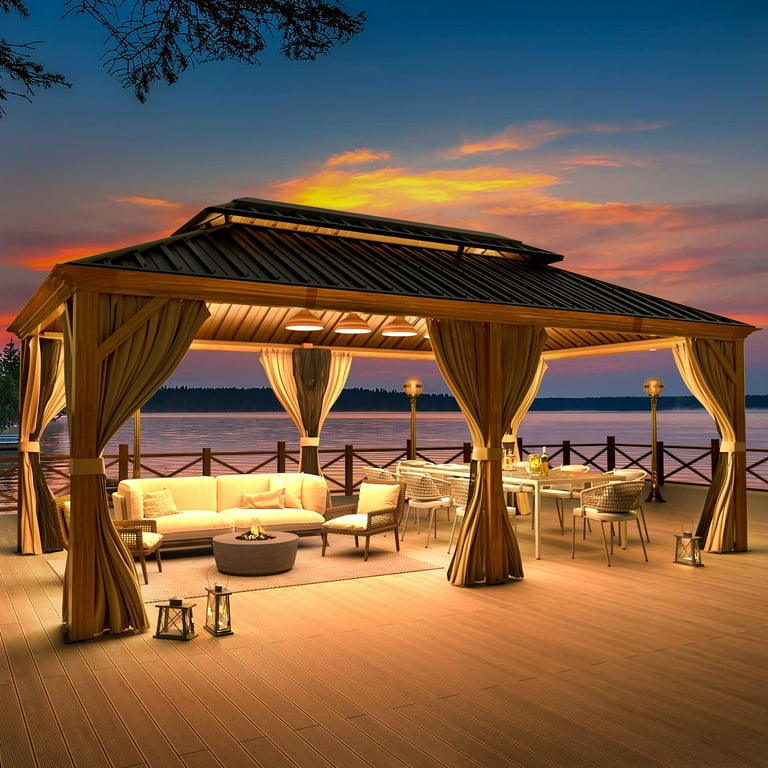The image depicts a serene, twilight scene of a large outdoor gazebo-style seating area situated on a wooden deck that extends over a body of water. The elegant structure features six tan and cream-colored curtains drawn back, which, if untied, would form fabric walls. Within the gazebo, a cozy arrangement includes a two-seat white sofa flanked by chairs, all centered around a round stone fire pit set on an area carpet. Nearby, a glass table is surrounded by seven chairs, with two wine bottles likely placed on it. The space is warmly illuminated by floor lamps and small lanterns strategically placed on the ground. Heaters are visible every few feet, ensuring the comfort of anyone present. The backdrop of the scene is a breathtaking sunset, casting hues of yellow, pink, and deepening blue across the sky, with glimpses of greenery peeking from above, enhancing the tranquil ambiance.